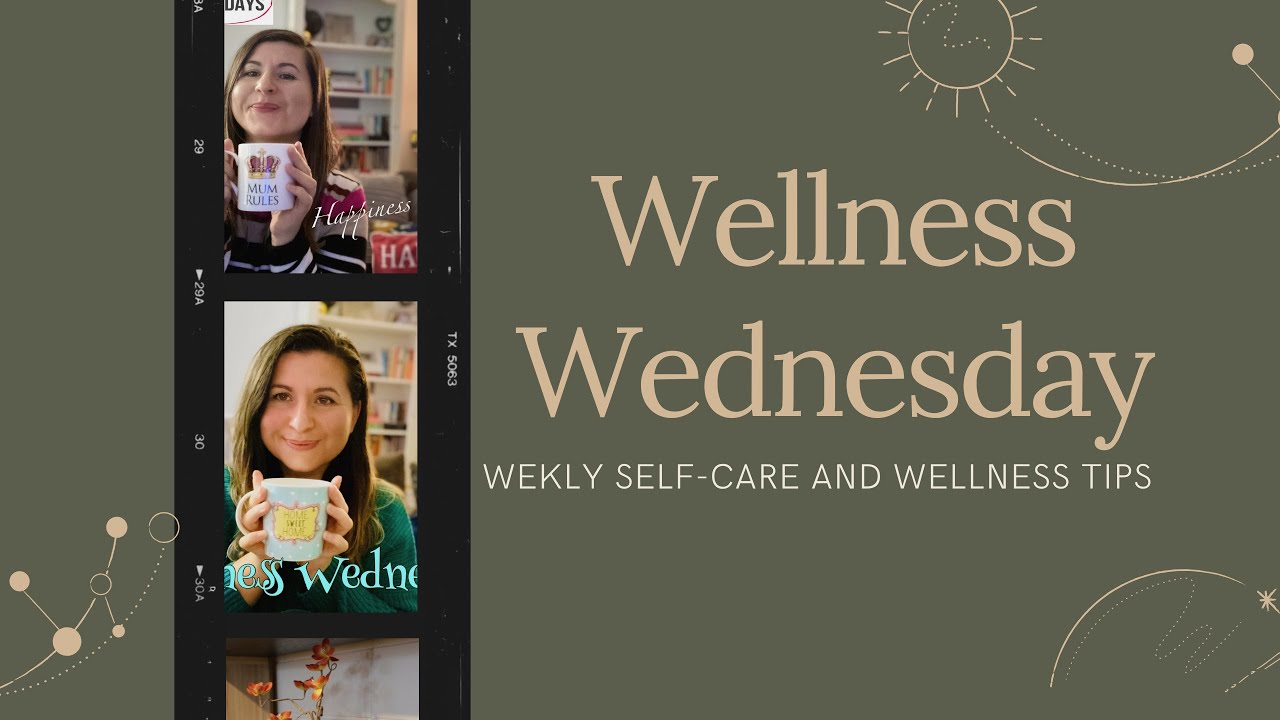The image features a rectangle with a military camouflage green background, reminiscent of the shades used in army uniforms. In the foreground, there is a vertical photo strip consisting of three images. The strip is bordered by black on both the left and right sides. 

At the top of the black border, the letter "A" is marked, followed by the numbers "29". A white triangle appears with the notation "20I" and a capital "A" inside it. Below this, the number "30" is inscribed, accompanied by another triangle with a "30A" marking. On the opposite side, the letters "TX" and the number "5063" are prominent in capital letters.

Within the images of the strip, a woman with brown hair appears repeatedly, each time holding a different mug. In the first photo, she holds a white mug adorned with the word "MUM" in uppercase letters beneath a crown graphic. The second shot shows her with a light teal-colored mug, however, part of the text on the mug is cut off, displaying only "E-S-S W-E-D-N," suggesting it might reference "Wednesdays." Adjacent to this mug, the phrase "Wellness Wednesdays" appears in a beige color. The final text reads "Self-Care and Wellness tips," but there is a typographical error where "weekly" is misspelled as "W-E-K-L-Y" instead of "W-E-E-K-L-Y."

The overall impression is of a serene yet attentive presentation focusing on self-care and wellness themes, curated with a mix of aesthetic and informative elements.